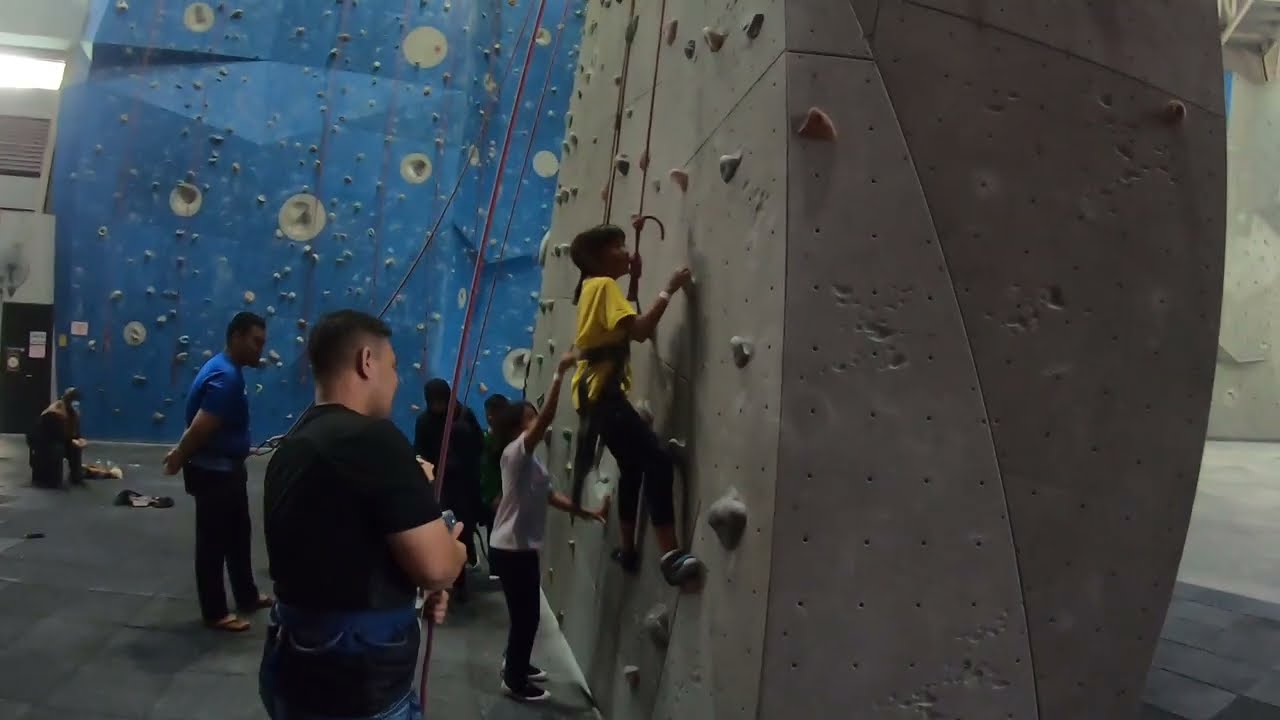The photograph captures an indoor recreational facility with two rock climbing walls, one prominently gray in the foreground and another light blue one in the background. Both walls are equipped with safety ropes. A young girl in a yellow T-shirt and black pants is climbing the gray wall, positioned a few steps up and facing to the right. Alongside her, slightly closer to the viewer, is a woman in a white T-shirt who appears to be getting ready to climb, and behind her is another girl in a purple shirt. Supervising the kids is a man with black hair, wearing a black T-shirt, closely monitoring with a safety line in hand, and another instructor in a blue T-shirt standing further back. There are additional shadowy figures near the walls, including one possibly kneeling at the far left edge of the image. The background is adequately lit, suggesting natural light from a window.